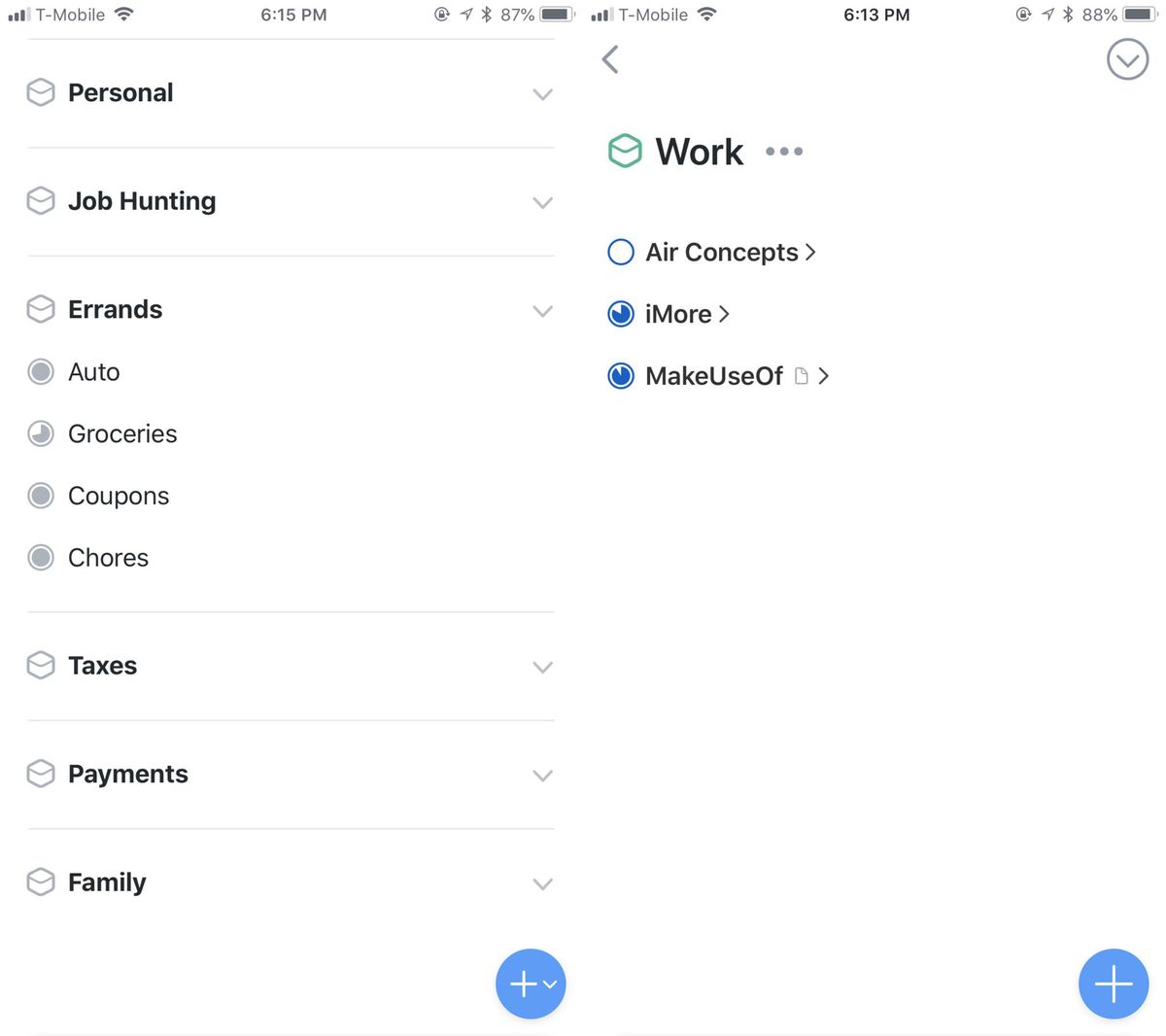The image consists of two side-by-side screenshots from a mobile app, each showcasing various menu elements and navigation options. 

In the left screenshot, a high-level menu is displayed prominently. This menu features several categories: Personal, Job Hunting, Errands, Taxes, Payments, and Family. Among these categories, only the Errands menu is expanded, revealing its sub-menu options: Auto, Groceries, Coupons, and Chores. A distinctive element in this screenshot is a large blue circular plus button situated at the bottom right-hand corner, suggesting the option to add new items.

The right screenshot focuses on a different part of the app, likely detailing one of the high-level menu options with an expanded sub-menu. The primary item visible is categorized under "Error Concepts," indicated by an arrow suggesting further expansion into a secondary menu. Below "Error Concepts" are two additional items: "I More" and "Make Use of," the latter accompanied by a small document icon. Similar to the left screenshot, a blue plus button is positioned in the bottom right-hand corner, hinting at a consistent design language across the app for adding new entries or items.

Both screenshots together provide a comprehensive look at the app's navigation interface, showcasing how users can explore and manage various categories and sub-categories.